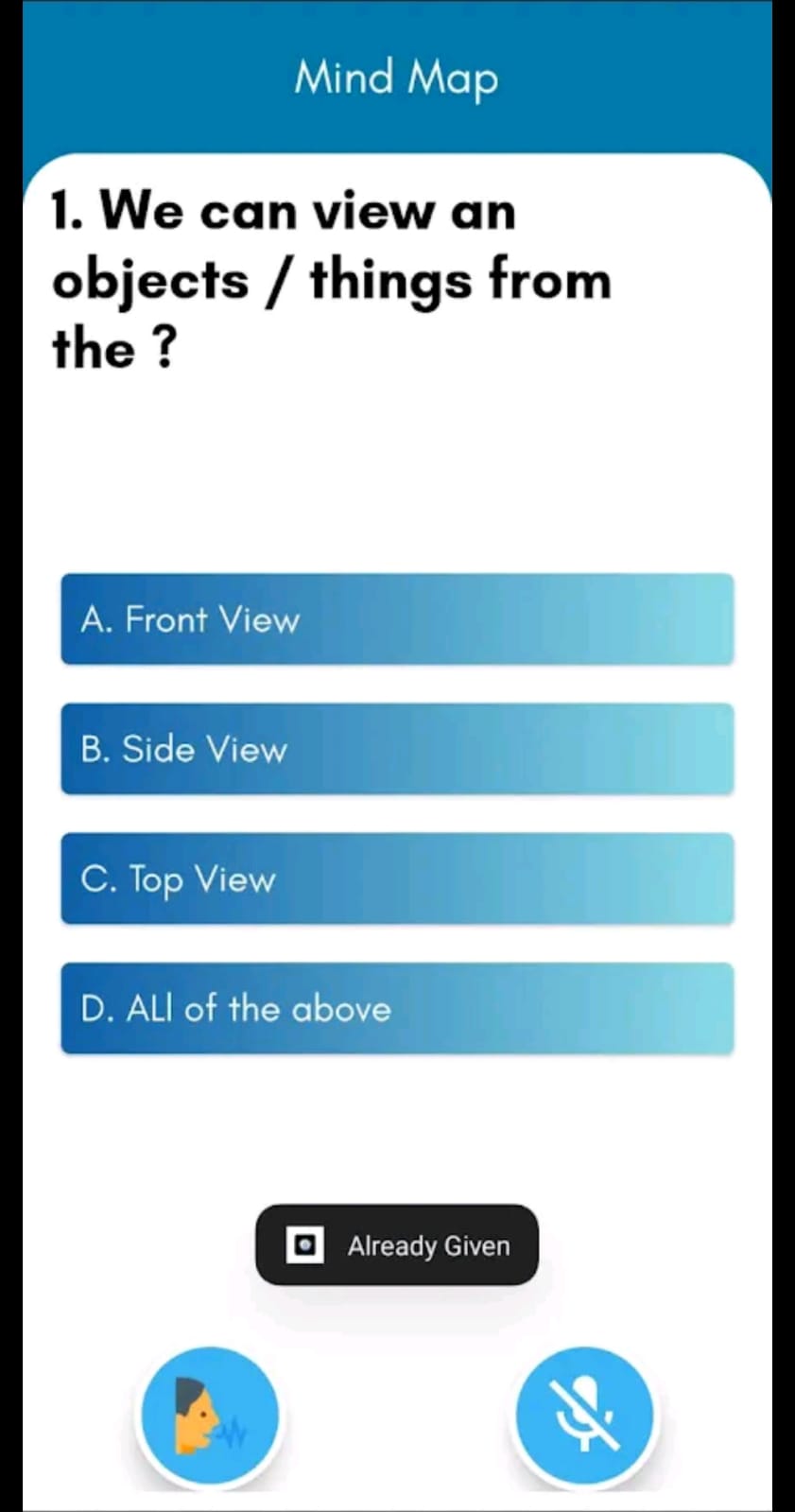The image features a medium blue top border with white text in the center that reads "Mind Map." The remainder of the image has a white background. Along the left and right sides of the image, there are two thin black lines. Within the white background, there is a text box that has the number "1" in black text. The accompanying text states: "We can view an object/things from the ?". Below this, there are four blue rectangles aligned horizontally. These rectangles transition from dark blue on the left to light blue on the right. Inside each rectangle, from top to bottom, the white text reads: "A. front view," "B. side view," "C. top view," and "D. all of the above." Underneath these options, there is an oblong-shaped black box containing the text "Already Given," which is aligned with a small white square to the left. Further down, on the left side, there is a light blue circle with an image of a person speaking. To its right, there is another light blue circle with a white microphone crossed out by a line, indicating it is muted.